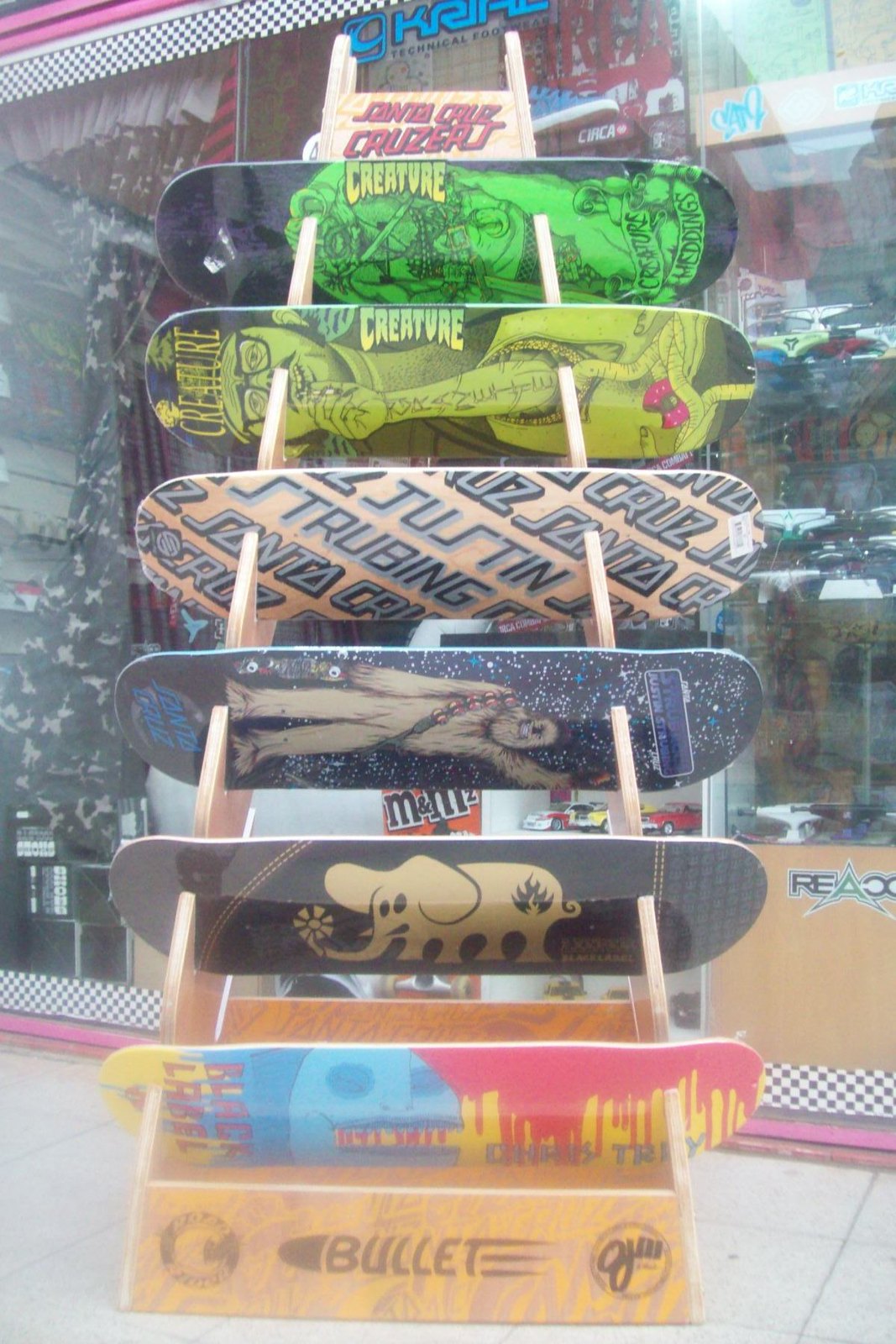In this vibrant color photo taken on a sunny day, we see an outdoor display of skateboard decks stacked on a wooden shelf in front of a storefront, which seems to cater to surf and skateboarding enthusiasts. The large glass window of the store provides a glimpse of the interior, adding a backdrop to the arrangement. The display shelf holds six distinct skateboard decks. The top deck features a black background with a neon green creature and the word "Creature" emblazoned on it. Below it, another "Creature" deck depicts a gentleman wearing glasses with a creature emerging from his chest. The third deck has an orange background with black letters spelling "Disturbing." The fourth deck is blue, showcasing a Wookiee-like figure. The fifth deck is black with a light yellow elephant adorned with flowers. The final deck at the bottom shows a monstrous face with blood-like elements in yellow and red. The diversity in colors and designs creates an eye-catching arrangement of the skateboard decks against the street-side store backdrop, inviting passersby to explore the shop.